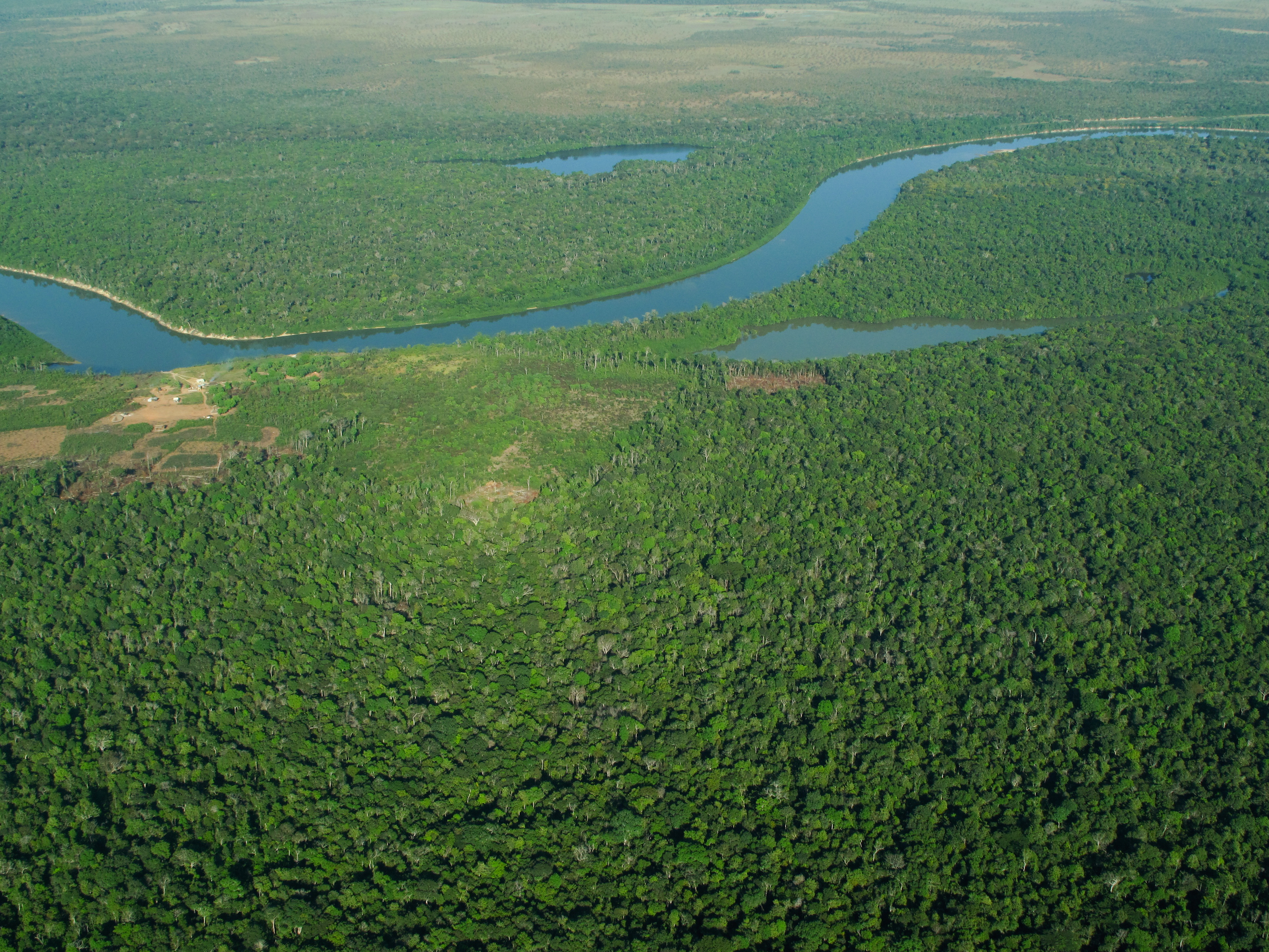This image captures a breathtaking aerial view of a lush, expansive jungle bisected by a winding, S-shaped river. The image is likely taken from about 100 feet above ground, offering an angled perspective down toward the river that meanders through the landscape. The river originates from the left side of the image, dips slightly downward, runs across the center, then curves upwards and exits to the right.

The terrain surrounding the river is predominantly dominated by dense green foliage, creating a vibrant display of natural beauty. In the upper third of the image, just below the midpoint, a small pond nestled among the greenery is visible, adding a serene touch. Further back, towards the upper part of the image, the lush green gives way to a more barren landscape, marked by brown and gray patches where the grass appears to have withered.

Below the main river, another smaller water body creates a tranquil pool, surrounded by a thin layer of green vegetation. This tributary also snakes through the forest, contributing to the intricate network of waterways within this verdant wilderness. The top and bottom sections of the image are engulfed in dense canopy tops, emphasizing the rich, unbroken stretch of jungle that spans the entire scene. On the far left, there might be hints of a farming field or another type of clearing, adding an intriguing contrast to the thick greens and waterways of the forest.